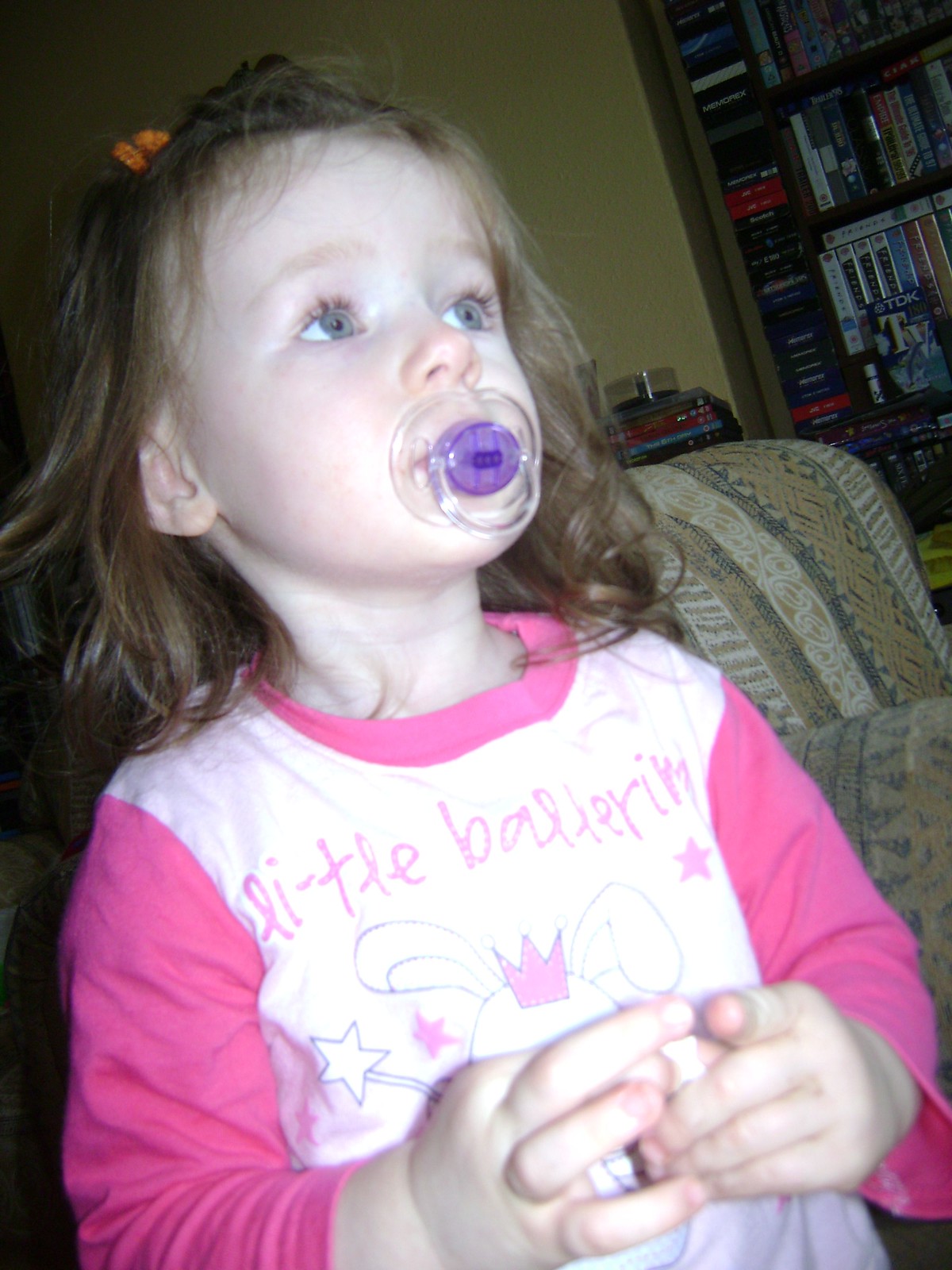The image is a horizontally oriented rectangle with natural borders, featuring a young Caucasian girl, likely around three to five years old. She has shoulder-length, slightly curly, red or orange hair pulled back with an orange barrette to the top left. Her vivid blue eyes gaze upward and to the right, and a purple pacifier rests in her mouth, giving her an imploring expression.

She is dressed in a long-sleeved or three-quarter sleeved white ringer shirt with pink sleeves and a pink ring around the neck. The shirt also features pink cursive writing that appears hand-drawn, spelling out "lit-tol b-a-l-t-o-l," accompanied by a hand-drawn pink and blue lined crown. Below this, a cartoon bunny is adorned with blue and pink stars.

The girl sits on a piece of woven furniture—possibly a couch, sofa, or small chair—patterned with stripes of white, gray, and yellow. A mustard-yellow wall stretches behind her and to the top right, complemented by a brown shelf to the right that holds a mix of DVDs and VHS tapes in various colors. There are about four horizontally aligned shelves with a mix of red, black, blue, white, and orange videos, capped with a yellow stripe at the bottom. Light illuminates her from an indeterminate source, hinting that the scene could be from any time between the 1970s and now due to the eclectic mix of color photography and objects in the room.